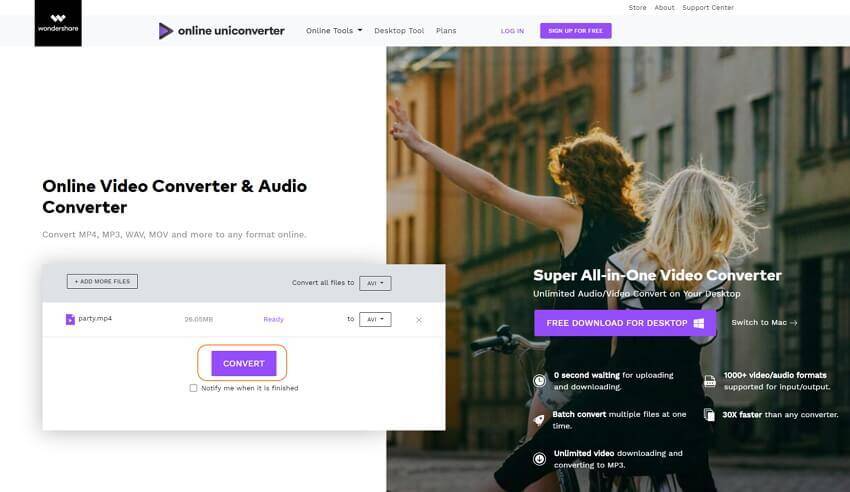The image showcases an online video and audio converter interface. In the top left corner, there is a black square containing a logo. To the right of this logo, the text "Online Converter" is displayed alongside a purple triangle. Further to the right, there are several categories written in purple, which include "Online Tools," "Desktop Tool," "Plans," and "Login," followed by a purple rectangle. This section is set against a light gray background.

Beneath this top section, on the left, the text "Online Video Converter and Audio Converter" is prominently displayed. Below this heading, there's a gray tab followed by four categories. Further down is a purple rectangle button labeled "Convert," outlined with a brown rectangular border. The majority of this section’s background is white, which continues around the entire interface.

On the right-hand side of the image, there is a picture of two people with long hair, viewed from behind, riding a bicycle. Above them are buildings in shades of brown, gray, and tan. Overlaying this image, the text "Super All-in-One Video Converter" is displayed. Below this text, there is an invitation to "Free Download for Desktop" in a light gray or light purple rectangle. At the bottom, there are five white options/buttons, three on the left and two on the right, completing the interface layout.